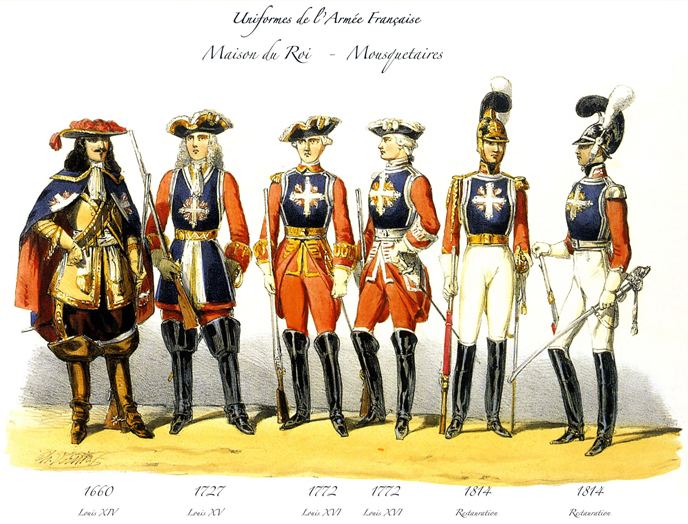The image is a detailed, color illustration depicting six soldiers from different historical periods of the French army. Arranged in a landscape orientation, the soldiers stand side-by-side on a tan-yellow base with a gray shadow behind them. The background is white, highlighting the vibrant uniforms.

At the top, in black cursive text, the title reads "Uniformes de l'armée Française." Below it is another line of French text, “Maison du Roy Mousquetaires.” Each soldier's attire represents a distinct era, marked by the dates at the bottom: 1660, 1727, 1772, 1772, 1814, and 1814.

The soldier on the far left, labeled 1660 Louis XIV, sports long dark hair, a mustache, an orange hat, a blue and orange cape, and a gold-colored uniform with baggy pants and high black boots. The next three soldiers, from 1727 Louis XV, 1772 Louis XVI, and 1772 again, are dressed in blue vests, orange pants and sleeves, and black tricorne hats. They all carry swords.

The final two soldiers, from 1814, are clad in blue chest armor, orange sleeves, white pants, and black boots. These soldiers wear helmets adorned with large feathers.

The detailed illustration shows a rich historical progression through the elaborate uniforms of these French military figures.